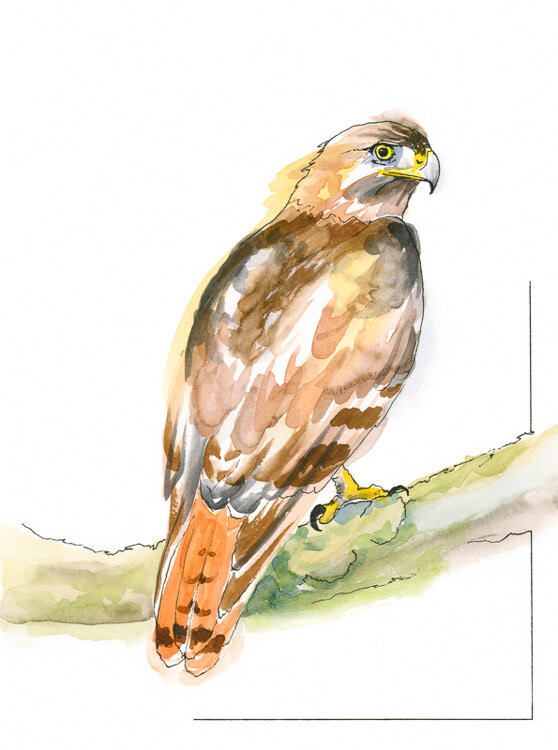This artwork is a detailed watercolor and ink painting of a bird perched on a green branch. The branch exhibits shades of green, ranging from light to dark, with subtle brown shadows at the bottom. The bird, possibly a hawk or eagle, is shown in right profile, showcasing a short, sharp white beak with a yellow nostril. Its eye features a yellow iris and a black pupil, framed by a slight gray area. The bird's plumage consists of varying hues, predominantly browns and tans with hints of yellow. Its tail feathers are adorned with orange and brown stripes. The bird's yellow legs are equipped with sharp black talons. The overall painting exudes a sense of meticulous detail, enhanced by the use of ink outlines and delicate watercolor smudging beyond the lines, emphasizing the textures and colors of the bird and branch.